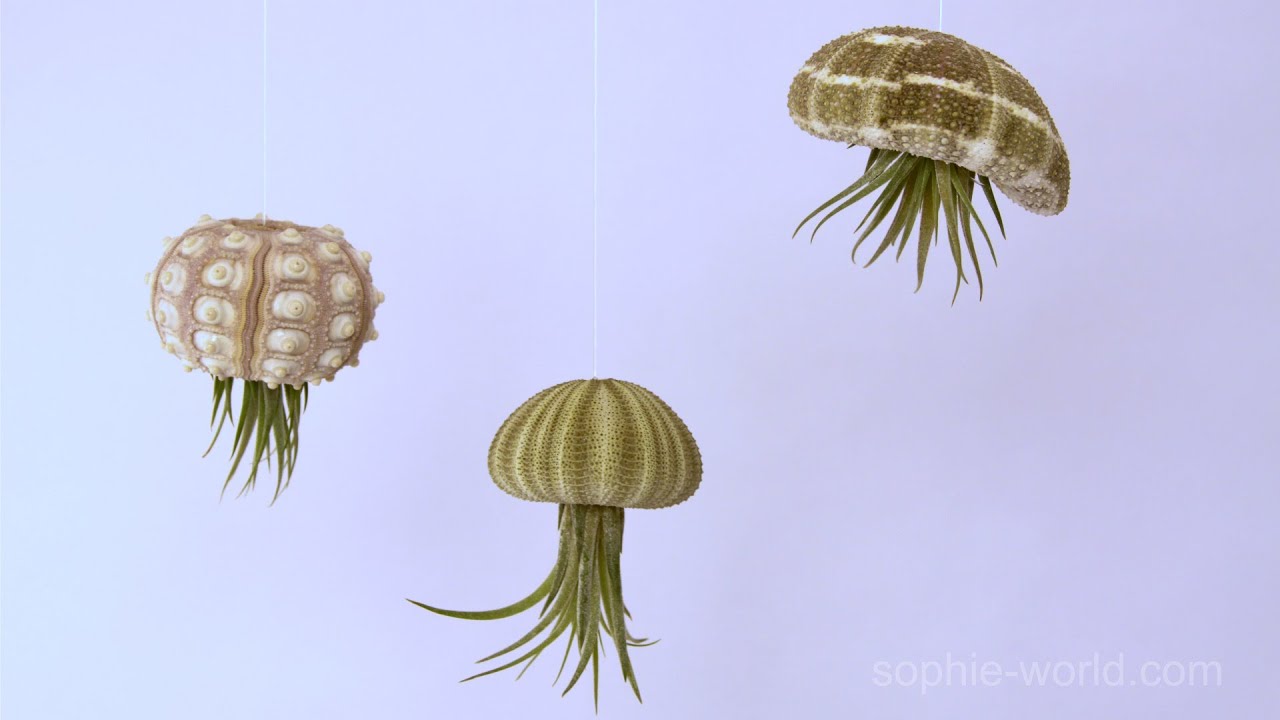In this photograph, we observe three captivating objects hanging from white strings against a light lavender backdrop. These objects resemble a creative blend of jellyfish and succulent plants, exhibiting photorealistic details. Each one possesses distinct features, yet they share common characteristics such as green tentacle-like growths extending from their bases.

On the far left, the object features a pink, bulbous top adorned with white bumps, reminiscent of a whimsical shell or sea creature's cap. In the center, a structure with a light brown and white, horizontally striped top hangs lower, presenting a jellyfish-like appearance with tentacle-like extensions. The object on the top right displays a unique green and white plaid shell-like top.

Additionally, the pale lavender background transitions to a lighter blue on the far left, creating a serene underwater-like atmosphere. The scene is complemented by the watermark "sophie-world.com" in the bottom right corner, indicating the source of this imaginative display.